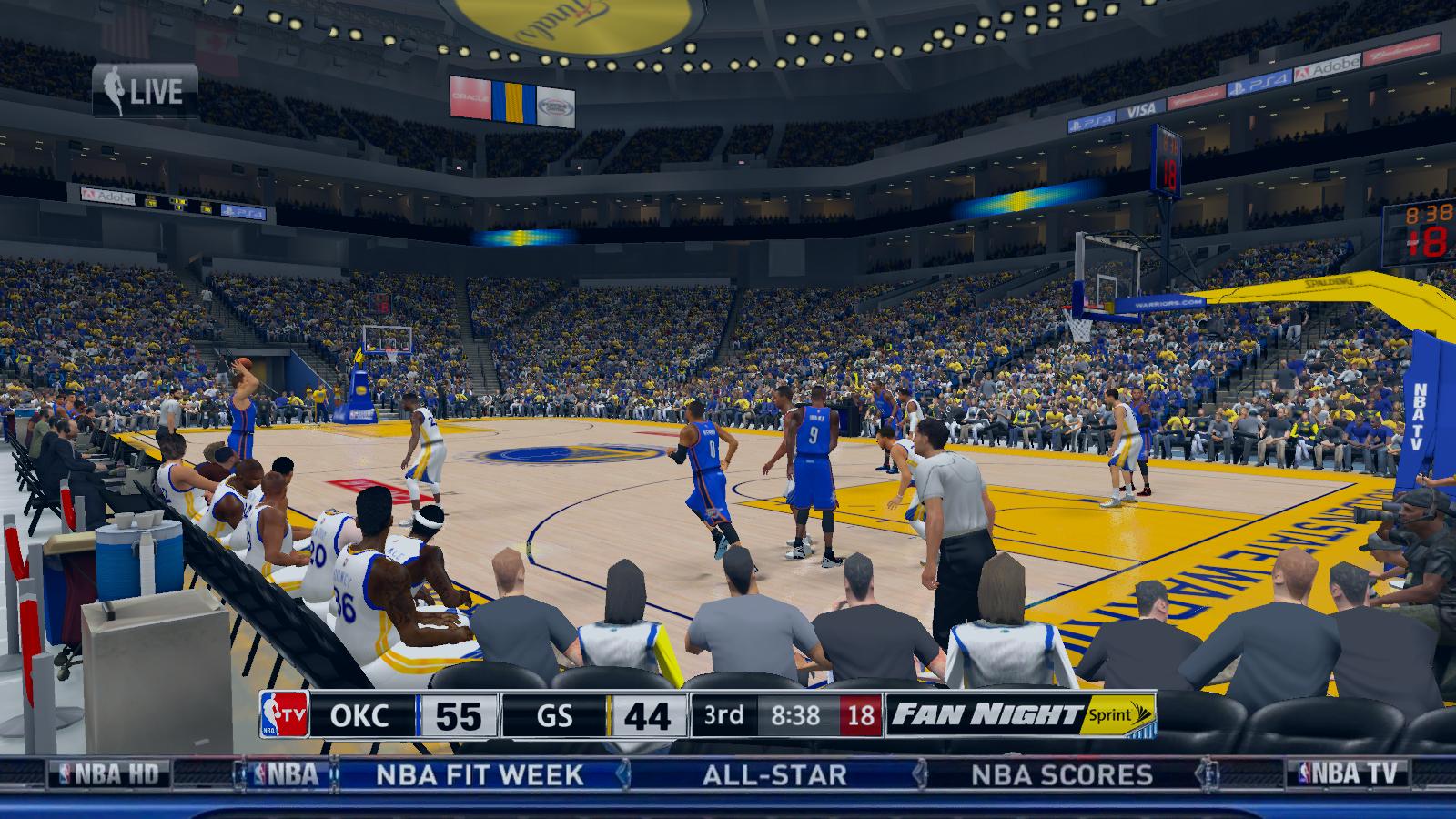The image showcases a vivid screenshot from an NBA video game, likely from the NBA 2K series, capturing an intense basketball match between the Golden State Warriors and the Oklahoma City Thunder. The Warriors, dressed in their distinctive blue uniforms, are up against the Thunder, who sport white uniforms accented with blue and yellow trim. The stadium is packed with enthusiastic fans, stretching from the top left to the top right of the background, creating a vibrant atmosphere. 

In the foreground, spectators are seated, while the Oklahoma City players are visible on the left, seated in chairs. A referee, clad in a white shirt and black pants, stands at the right edge of the court. Central to the scene, an Oklahoma City Thunder player holds possession of the ball, poised to make a play. The scoreboard at the bottom of the screen reveals that the Thunder are leading with a score of 55 to the Warriors' 44 in the third quarter. Additionally, a smaller banner above the scoreboard indicates it's "Fan Night Sprint."

Prominent banners running along the bottom of the screen boast the "NBA HD" logo, as well as references to "NBA Fit Week," "All-Star," "NBA Scores," and "NBA TV," affirming the game's official NBA branding and highlighting the immersive experience of the video game.